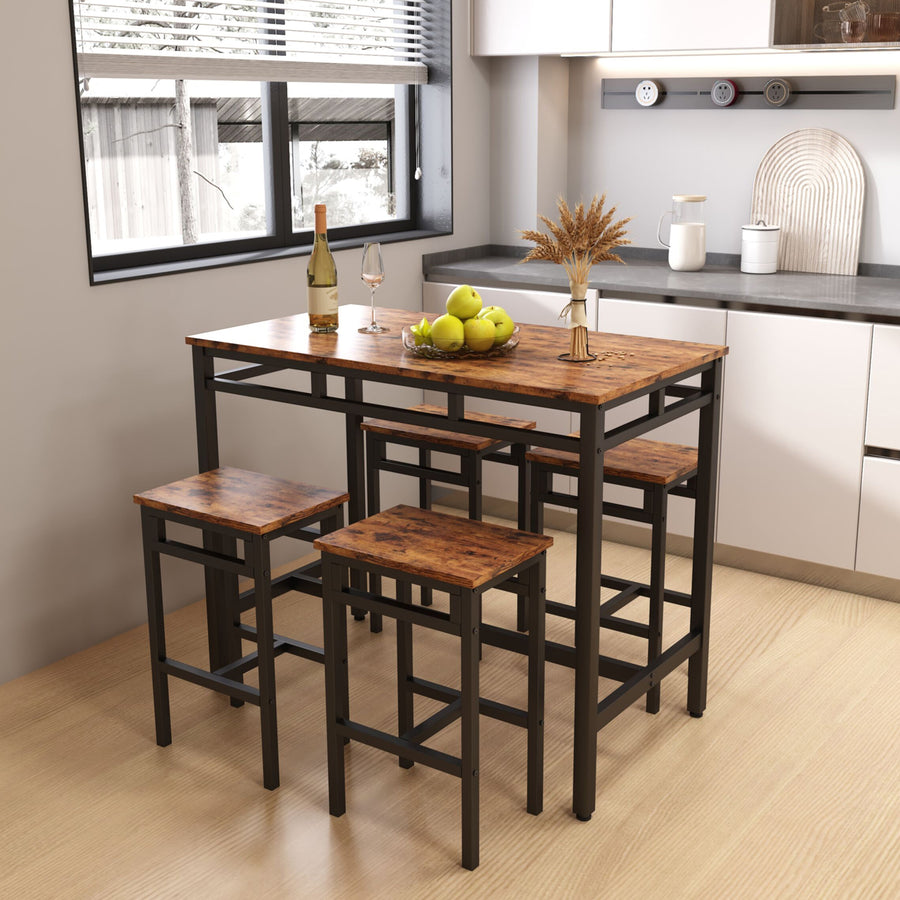The photo depicts a dining area within a kitchen, characterized by a modern and cohesive aesthetic. Dominating the scene is a long, narrow rectangular table with a natural wood tabletop marked by a dark grain, supported by a sleek black metal frame. Accompanying the table are four backless bar stools, neatly tucked underneath, that share the same wood and black metal design.

The kitchen boasts white walls, white cabinets, and a gray countertop that contrasts with the light wood flooring. A window to the left, framed in black with half-open white blinds, offers a glimpse outside where metal structures and a pole are visible.

On the table, a glass bowl filled with green apples sits beside a bundle of dried wheat standing upright, while a bottle of wine and a wine glass complete the tableau. The countertop area and some decorative white containers can be seen in the background to the right, adding to the kitchen's clean and elegant look.